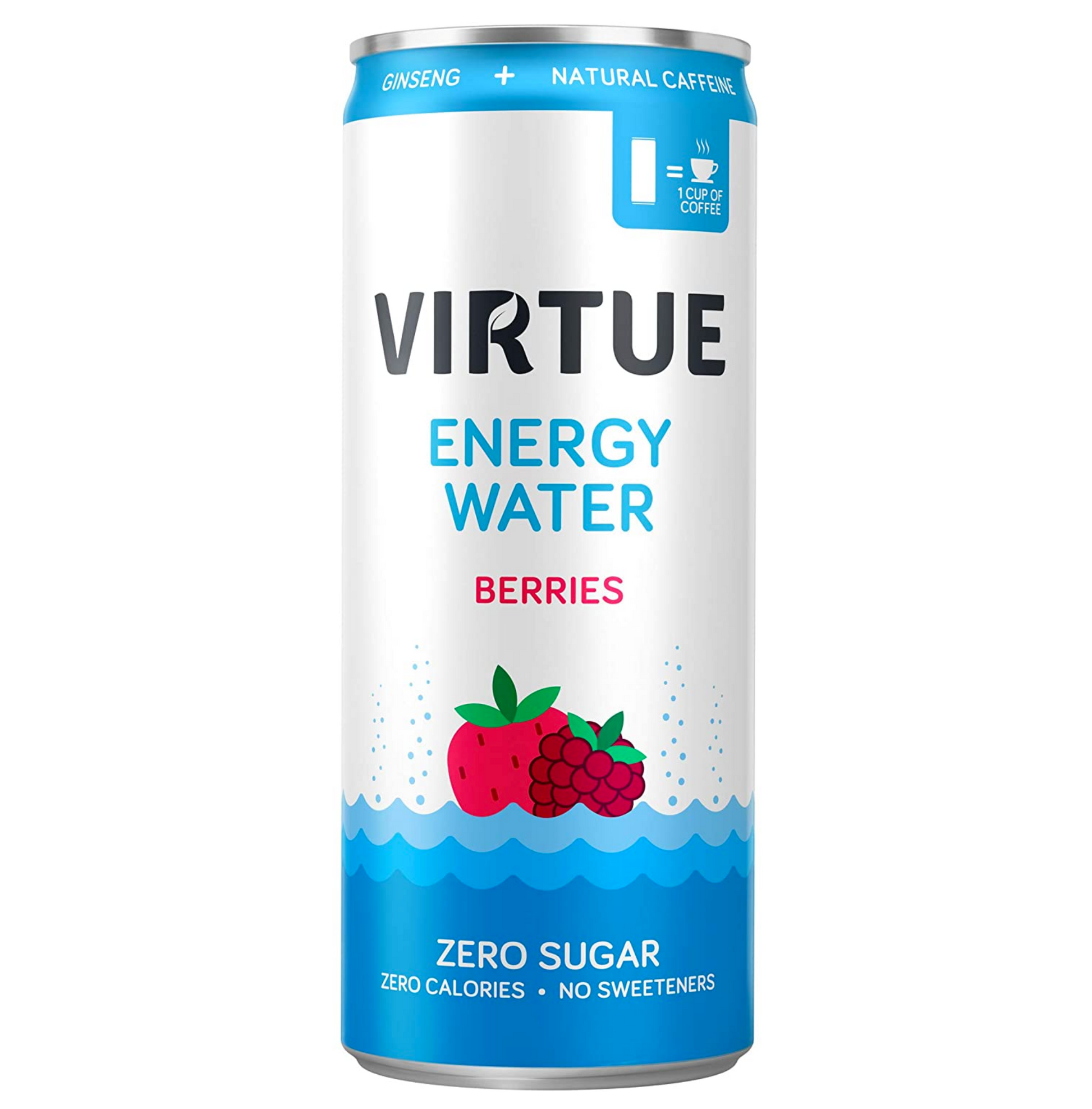This image is a detailed close-up of a slim can of Virtue Energy Water, rendered in either a highly realistic photograph or a 3D rendering. The can features a silver top and bottom with a label covering the middle. At the top of the label is a narrow blue strip with white text that reads "ginseng + natural caffeine." Below this is a small blue tab stating "one can = one cup of coffee." The brand name "Virtue" is prominent in black capital letters on a predominantly white or silver background, with the hole in the "R" cleverly designed as a leaf. Beneath the brand name, "energy water" is written in blue text, followed by the flavor "berries" in red. The can's lower section illustrates a strawberry and a raspberry floating on water, which is depicted in three stripes of light blue, medium blue, and dark blue. Bubbles rise up from the water, and at the bottom, in white text on the dark blue part, it reads "zero sugar, zero calories, no sweeteners." The overall design features a harmonious blend of silver, blue, and red colors, emphasizing its natural ingredients and health benefits like ginseng and natural caffeine.